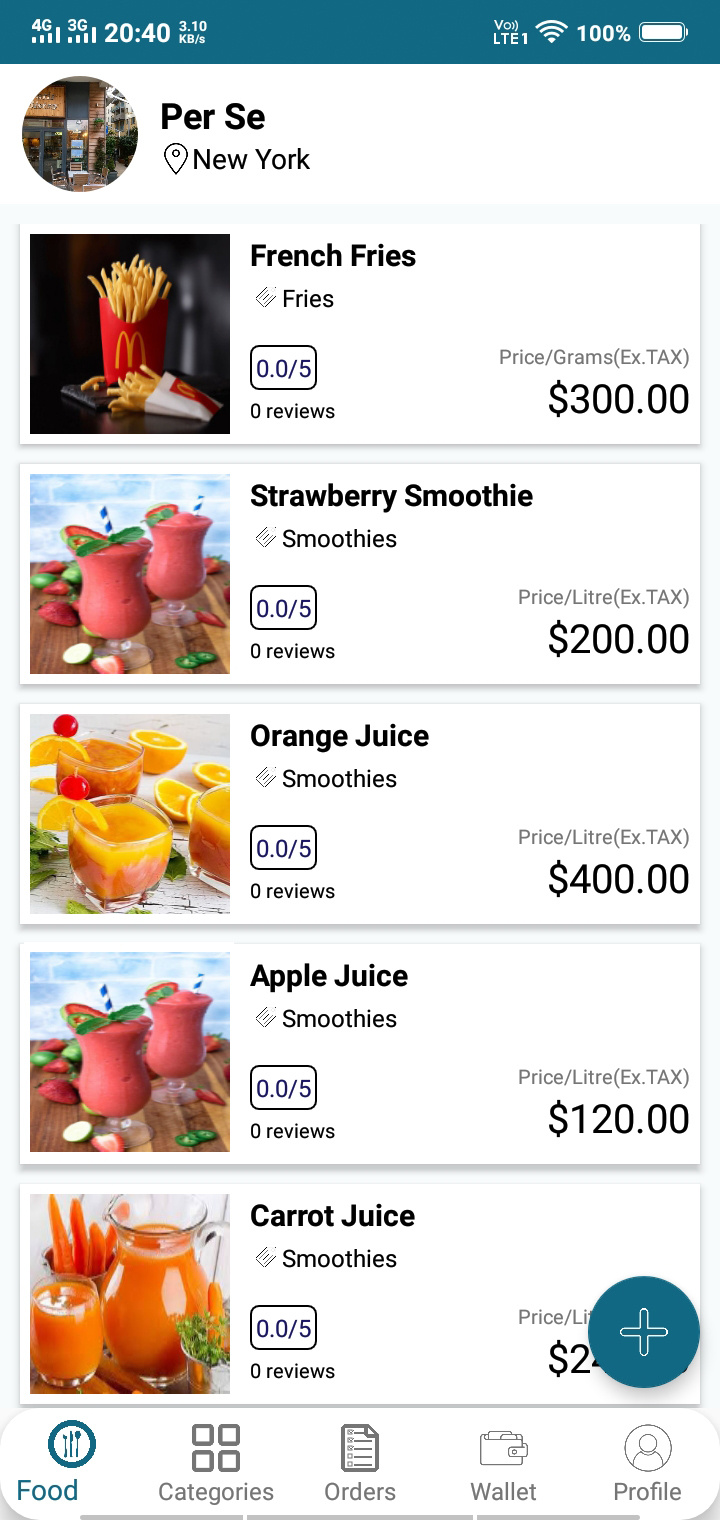Here is a cleaned-up and detailed caption for the described image:

---

The image showcases a mobile application interface on a white background. The top section features a green border, where the right side displays battery status, Wi-Fi connectivity, and cellular signal icons, indicating 4G and 3G connections. The current time is shown as 20:40.

Below this top section, there is substantial white space leading to the main content area on the left side of the screen. Here, a circular profile photo is labeled "Prse," with "New York" written underneath it, accompanied by a location pin icon, suggesting the place or current location.

Further down, a series of rectangular sections display various food items and their details. The first rectangle on the left shows an image of McDonald's fries with a description on the right reading "French fries price grams $300." Following this, subsequent rectangles present additional food items with both images and prices:

- Two strawberry smoothies in glasses with a price of $200.
- Orange juice priced at $400.
- Apple juice for $120.
- Carrot juice, though partly covered, indicating a similar display.

At the bottom of the interface, a navigational menu consists of several buttons labeled "Food," "Categories," "Orders," "Wallet," and "Profile." The overall color scheme of the app is predominantly white, interspersed with colored images and price tags for clarity and visual appeal.